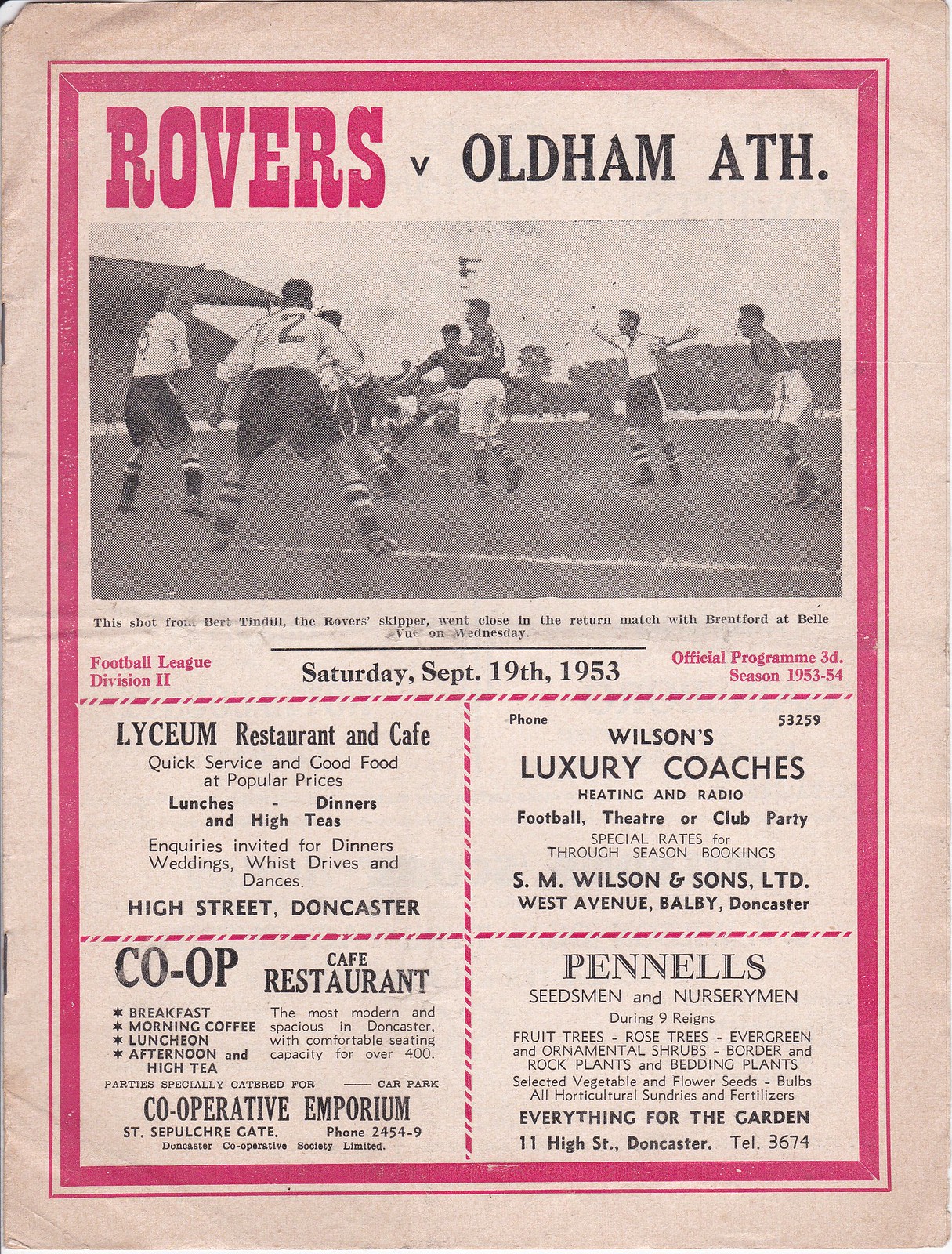This image is of the weathered cover of an old football program for a Football League Division Two match between Rovers and Oldham Athletic, held on Saturday, September 19, 1953. The off-white background is framed by a red rectangular border, and text in red and black reads "ROVERS V OLDHAM A." The program features a black and white picture of six to eight football players on the pitch, some with outstretched arms and others in action, with numbers visible on their backs, such as 2 and 5. Beneath the image, difficult-to-read caption text appears. Further down, it states "Football League Division Two," the date of the match, and mentions it is an official program for the 1953-1954 season, priced at 3D. At the bottom, there is a matrix of four advertisements: Lyceum Restaurant and Cafe, Wilson's Luxury Coaches, TV and Radio, Co-op Cafe Restaurant, and Pennell's Seedsmen and Nurserymen.